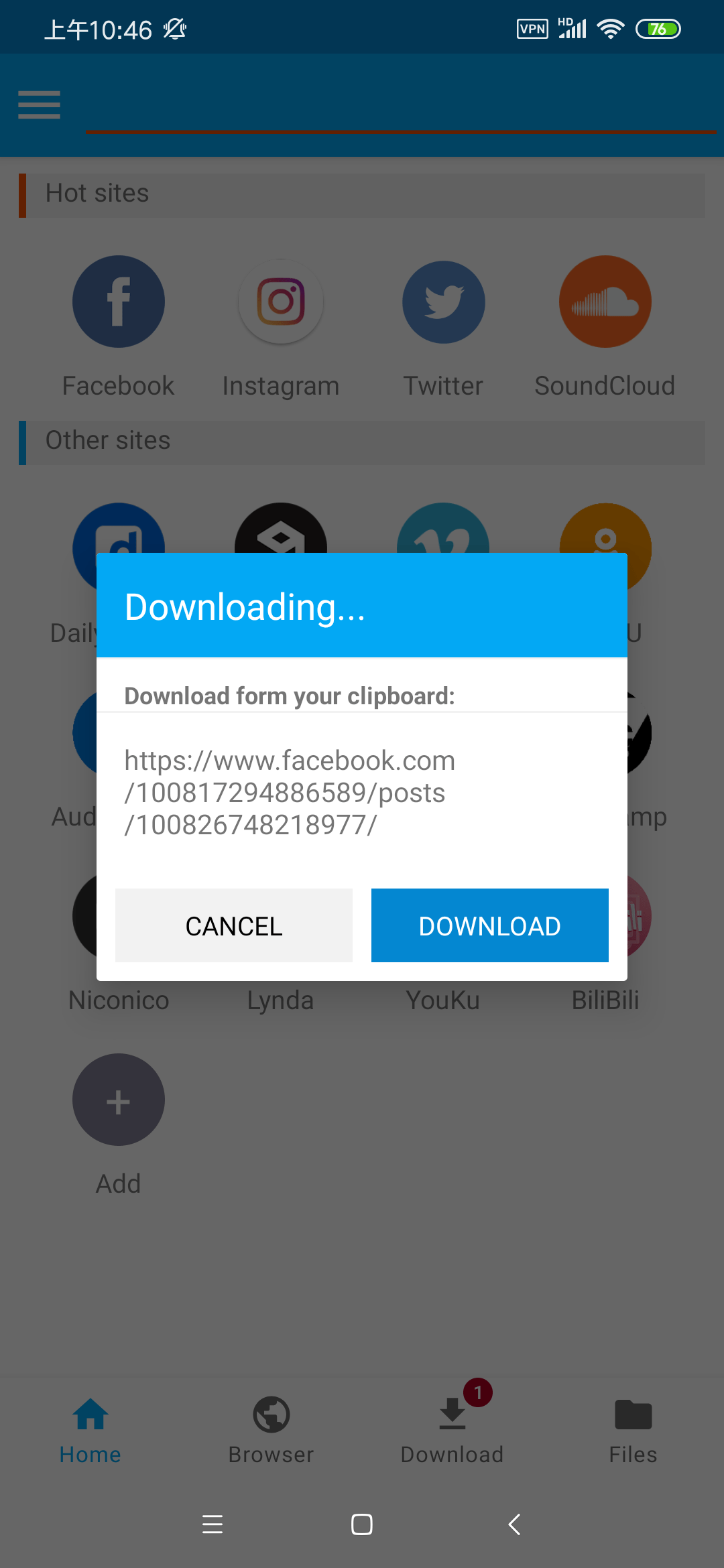A detailed description of the cell phone screen image:

The cell phone screen features a variety of icons situated along the status bar at the top. From left to right, several icons are present, which are not easily identifiable. The time displayed is 10:46, and a bell icon with a diagonal line through it indicates there are no notifications. Additional icons include a VPN indicator, HD signal, cell signal bars, Wi-Fi signal bars, and a battery icon showing 76% charge in green.

The screen is overlaid with a semi-transparent gray layer. Superimposed on this overlay is a rectangular dialog box with a horizontally elongated shape. The top strip of this dialog box is blue and contains the text "Downloading..." in white. Below this, on a white background, is a message in black text that reads: "Download from your clipboard: https://www.facebook.com/100817294886589/posts/100826748218977/".

At the bottom of the dialog box are two buttons: a gray "Cancel" button with black text, and a blue "Download" button with white text.

In the background, partially covered by the overlay and dialog box, are the main contents of the cell phone’s home screen, which showcases four rows of app icons.